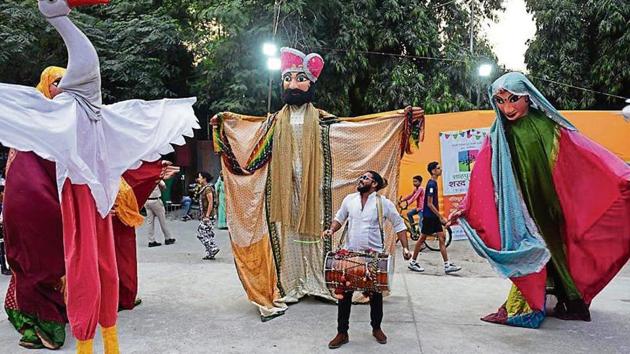This vibrant outdoor festival scene captures an eclectic mix of cultural and fantastical elements against a bright and lively backdrop. At the center of the image stands a man with his hair pulled back in a bun, sporting a white shirt, black pants, and brown shoes. He has a drum horizontally strapped to his front and is staring upwards, accentuated by glasses and a beard. Surrounding him are towering figures, each about 10 feet tall, dressed in elaborate costumes. To his right, a woman on stilts wears a green-pink gown and a blue headdress, evoking an Indian or Persian aesthetic. Further right, another giant figure dons a purple headdress and a richly decorated Persian-style outfit. To his left, a whimsical character dressed as a large white bird with outspread wings and a red nose appears, though its head is partially out of frame. In the background, people walk by, including a child on a bike, against a yellow wall partition adorned with posters. Strings of lights hang from poles, and trees can be seen in the distance, completing the festive and enchanting tableau.